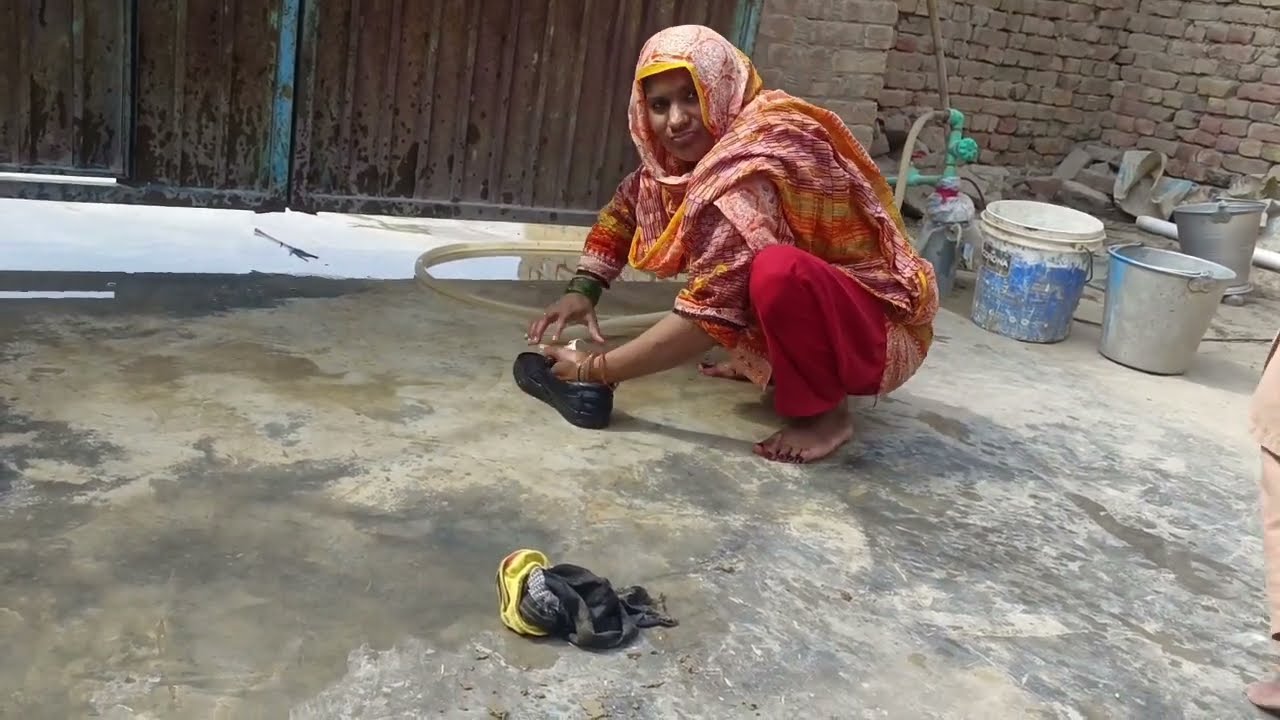In this detailed image, we see a Middle Eastern woman dressed in vibrant traditional attire, crouching barefoot on a concrete ground. She wears red pants and a multi-colored tunic in shades of pink, orange, and yellow, paired with a matching headscarf that covers her head but not her face. The woman is squatting down, holding a black shoe in her left hand, her right hand poised to grab it, suggesting she might be cleaning or polishing it. The surrounding scene includes a stone-paved area marked with water stains and some scattered pieces of clothing, including what appears to be a child's shoe and socks. Behind her, there are two buckets—one a dirty blue with white and blue paint markings, the other a light gray—positioned next to a primitive brick building. To her right is a wooden or metal gate with more water on the ground, indicating a chore-related activity. The woman is looking towards the camera, adding a sense of engagement to the scene.